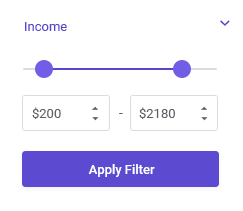This screenshot captures a portion of a form interface. At the top left, the label 'Income' is prominently displayed in purple text. Adjacent to it on the right is a down arrow icon, suggesting the option to collapse this section. Directly below, there is a horizontal slider with two circular handles—one nearer to the left end and the other closer to the right end of the purple line.

Further down, there are two monetary input fields. The field on the left is filled with the amount $200, while the one on the right displays $2,180. Each field is accompanied by two small arrows beside the number, allowing for incremental adjustments up or down.

Beneath these input fields is a bold purple button labeled 'Apply Filter' in white text. The entire section rests on a clean, white background which enhances the readability and organization of the interface elements.